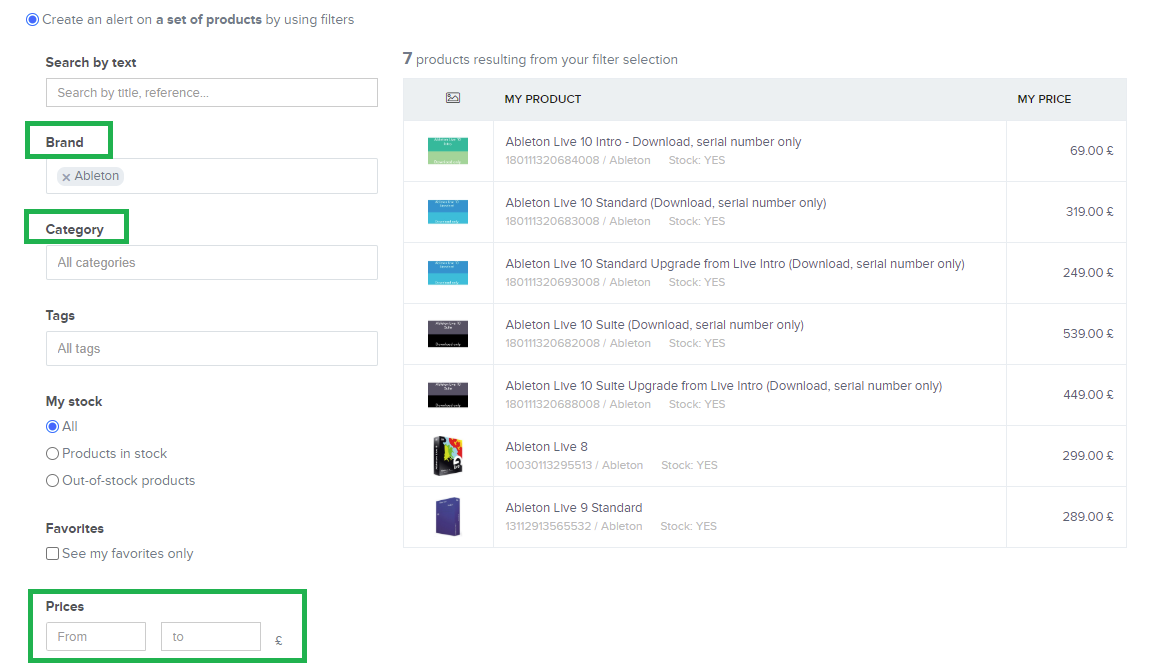**Detailed Caption:**

The image is divided into two columns. The narrow left-hand column occupies roughly one-third of the image, whereas the wider right-hand column takes up about two-thirds. In the upper left corner of the image, there is a blue dot encircled by a blue outline along with the text, "Create an alert on a set of products by using filters."

On the left-hand column, several search filters are described sequentially. 

1. **Search by Text**: A rectangular search box appears here.
2. **Search by Title, Reference**: This is another instance of a search filter.
3. **Brand**: This has a green outline, and the underlying box contains the text "Ableton," which is grayed out with an 'X' next to it.
4. **Category**: This filter is also highlighted with a green outline, displaying "All Categories" in the box beneath it.
5. **Tags**: This is denoted by "All Tags" in the box below the term.
6. **My Stock**: This section has a selected option marked with a blue dot labeled "All." Below it, there are two open dots labeled "Products in Stock" and "Out of Stock Products" respectively.
7. **Favorites**: This filter includes a checkbox next to the statement "See My Favorites Only."
8. **Prices From**: This section contains two boxes side-by-side, the first one for the minimum price and the second for the maximum price.
 
The wider right-hand column indicates the result of the search filters, displaying the text "7 products resulting from your search filter." Below this, the column is structured to exhibit product details and includes headings or icons for "Image," "My Product," and "My Price."